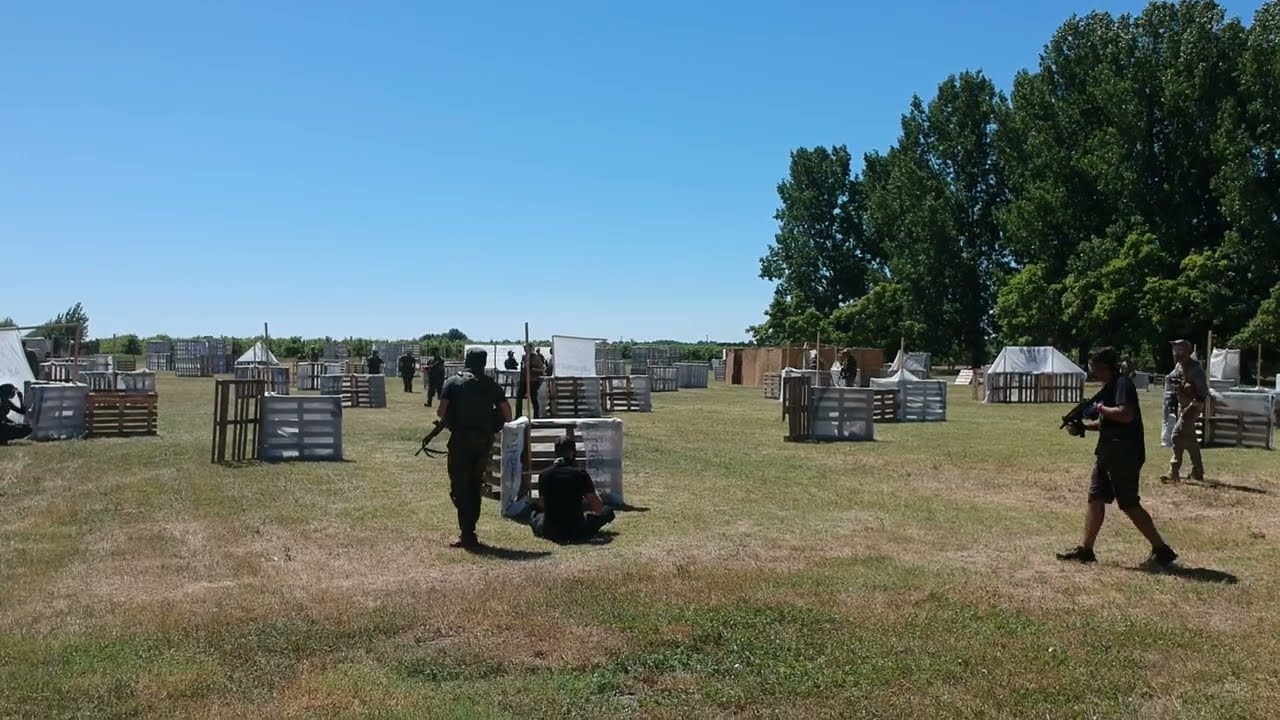In this detailed outdoor photograph, a group of individuals, clad in dark attire that resembles military or tactical gear, are engaged in what appears to be a paintball game. They are equipped with paintball guns, some resembling machine guns, and wearing protective masks and helmets. The expansive field is dotted with numerous wooden pallet barriers set up as makeshift cover stations. Some of the barriers are transformed into small tent-like structures using white cloth as roofs.

In the foreground, one man is seen sitting cross-legged in front of one of these pallet constructions, while others are either walking around or crouching behind the barriers, seemingly in a relaxed state, indicating a possible break or strategy session. The scene is well-lit by the bright sun, casting clear blue skies overhead. To the right, a line of tall trees provides a natural boundary to this large, open field, which is lush with green grass and scattered with pallet stations every few feet, providing ample cover and strategic points for the paintball participants.